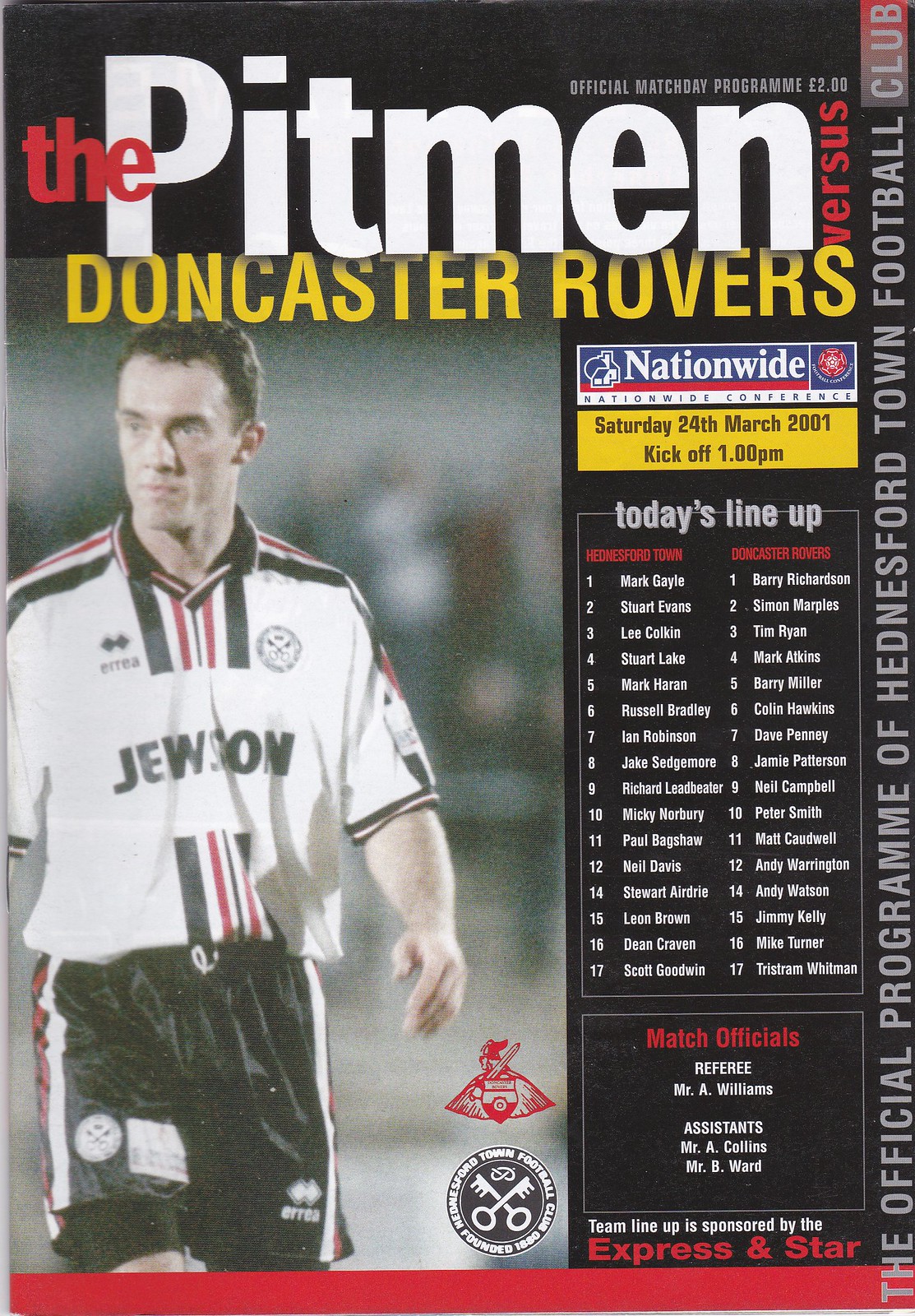This image is the cover of a soccer program for the match between The Pitmen and Doncaster Rovers, held on Saturday, 24th March 2001, with kickoff at 1 p.m. The cover features a photograph of a soccer player wearing a white jersey with red and black stripes along the shoulders and front. The player's name appears to be Jewson. He has short cropped hair and is wearing black shorts. 

To the left of the player, there's the logo of the soccer team, depicting a Viking holding a sword in front of a shield. Another round logo nearby reads "Hedonistford Town Football Club, founded 1880." At the top of the page, there's a black border extending down the right side, which contains the text "The Pitman versus Doncaster Rovers."

Below the main image, a yellow text box announces the sponsorship of the Nationwide Conference and details of the match. There's another text box over a black background that lists "Today's Lineup," displaying 17 players from each team, followed by the names of the match officials, including the referee and assistants. The team lineup is sponsored by Express and Star. Additionally, the phrase "The official program of Hedonistford Town Football" runs vertically along the right-hand side. 

The program is priced at two pounds, stating "Official Match Day Program" in the upper right corner. The text "The Pitman" stands out in yellow and red, while "Doncaster Rovers" is also highlighted in yellow. The bottom left corner bears a logo with crossed keys, possibly referencing another sponsor, ARIA (E-R-R-E-A), affixed to the player's jersey. Overall, the program cover encapsulates a vintage feel, characteristic of an early 2000s sports event.